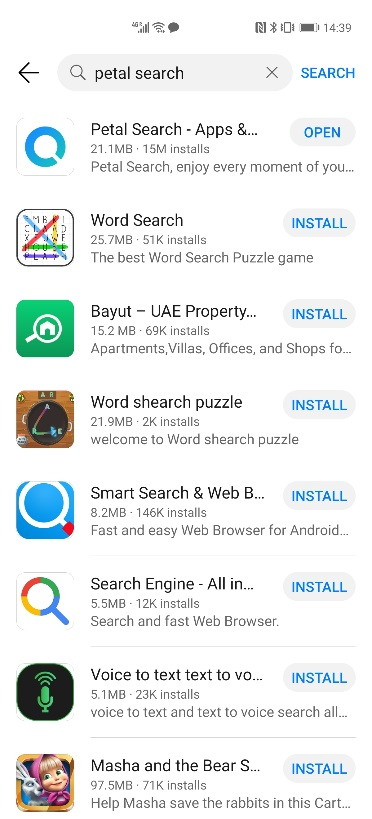Screenshot of a website depicting a search results page. At the very top of the screen, the status bar displays various icons such as Wi-Fi and signal strength indicators, along with the time set in a 24-hour format: 14:39. 

Immediately below the status bar is a search bar where the user has typed in "P-E-T-A-L search." To the left of the search bar, there is a back arrow icon, and to the right, a search icon. 

The main content of the screen consists of a list of search results. The first option is "Petal Search Apps," which appears to be a category or recommendation. Below that are individual search results with options to install each one:

1. **Word Search**
   - Option to install
   - Information on storage space required and the number of installs.
   - Related tags.

2. **Word Search Puzzle**
   - Option to install
   - Details on size and the number of downloads.
   - Associated tags.

3. **Smart Search and Web**
   - Option to install
   - Specifications on storage and installations.
   - Related tags.

4. **Voice to Text, Text to Voice**
   - Option to install
   - Data on required space and install count.
   - Related tags.

5. **Masha and the Bear**
   - Option to install
   - Information on space usage and number of installs.
   - Related tags.

Each app's title is displayed in bold letters, with details such as storage requirements and the number of installs shown in regular font beneath the title. The tags related to each app are also visible, providing additional context and relevancy to the search results.